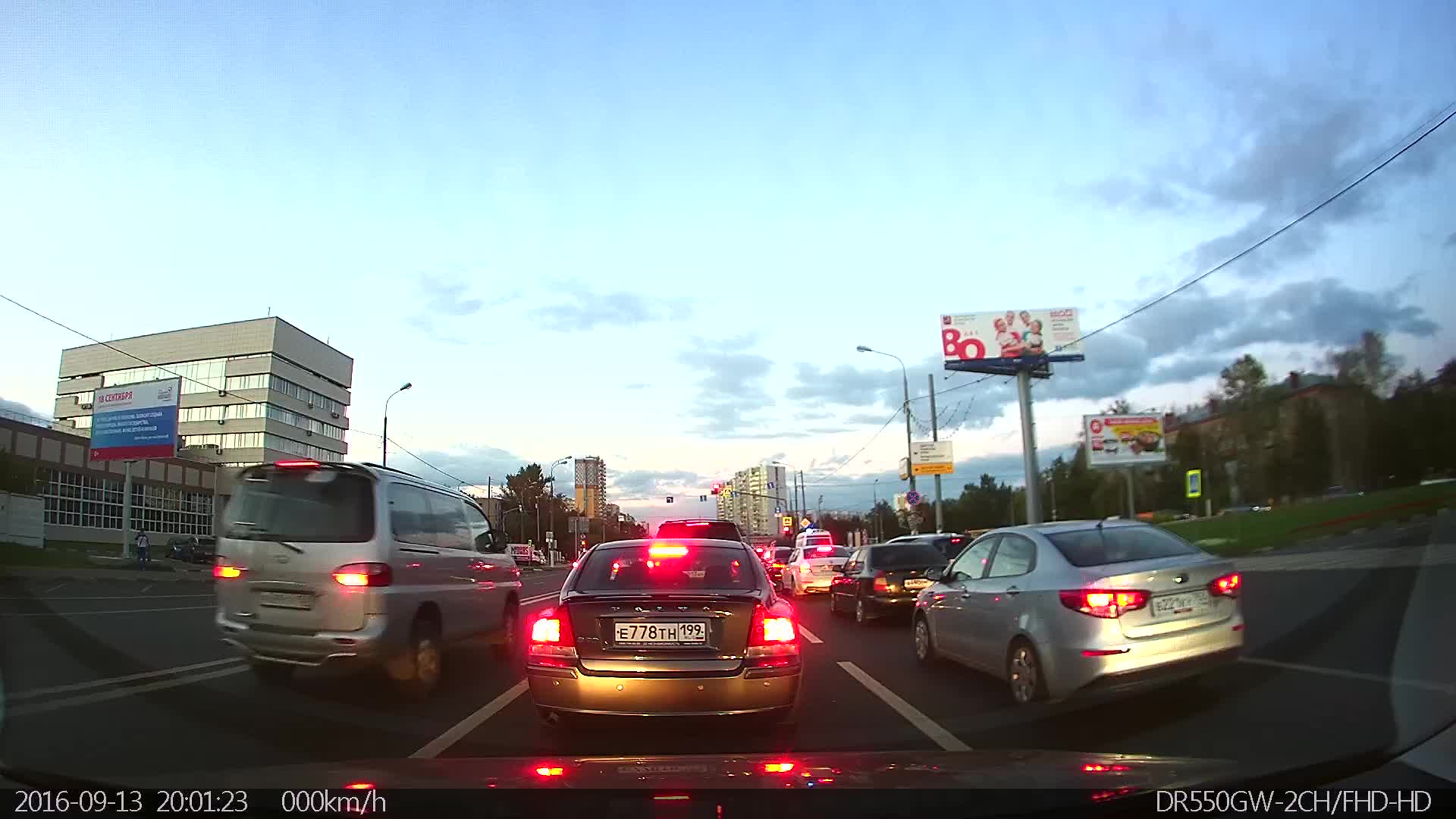This high-quality dash cam photograph, dated 2016-09-13, features a bustling urban scene. Stamped on the image are the time and a string of alphanumeric characters. Dominating the foreground is an olive green car, accompanied by a silver van and a silver sedan nearby. Several other vehicles are also visible ahead.

To the left, a large gray building stands prominently. In the parking lot, a red, white, and blue sign is noted, while to the right, a white billboard with bold red font captures attention. Multiple other billboards and road signs pepper the horizon, alongside a stoplight ahead.

Overhead, power lines crisscross the scene, while the pavement below is marked with white lines. The sky above shows a partial glimpse of a slightly darkened blue sky, peppered with gray clouds, adding a subdued contrast to the otherwise vibrant urban environment.